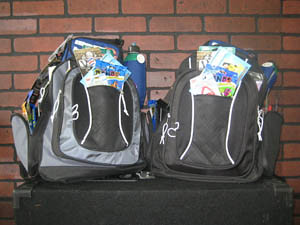The photograph features a dark red brick wall in the background with dark brown grout, suggesting an interior setting. Dominating the foreground is a black rectangular table or trunk, spanning nearly the width of the image and situated just above the bottom edge. Placed on this table are two backpacks, both overflowing with contents. The left backpack is predominantly gray with black outlines, featuring a pocket containing a blue thermos with a green lip and silver cap. The right backpack is entirely black, adorned with two vertical white lines. Both backpacks are from the same maker, evidenced by similar designs and markings. They are stuffed with various items, possibly books or papers, adding a sense of chaotic fullness. Strings or straps, potentially from headphones, also dangle from the bags, contributing to the cluttered appearance.